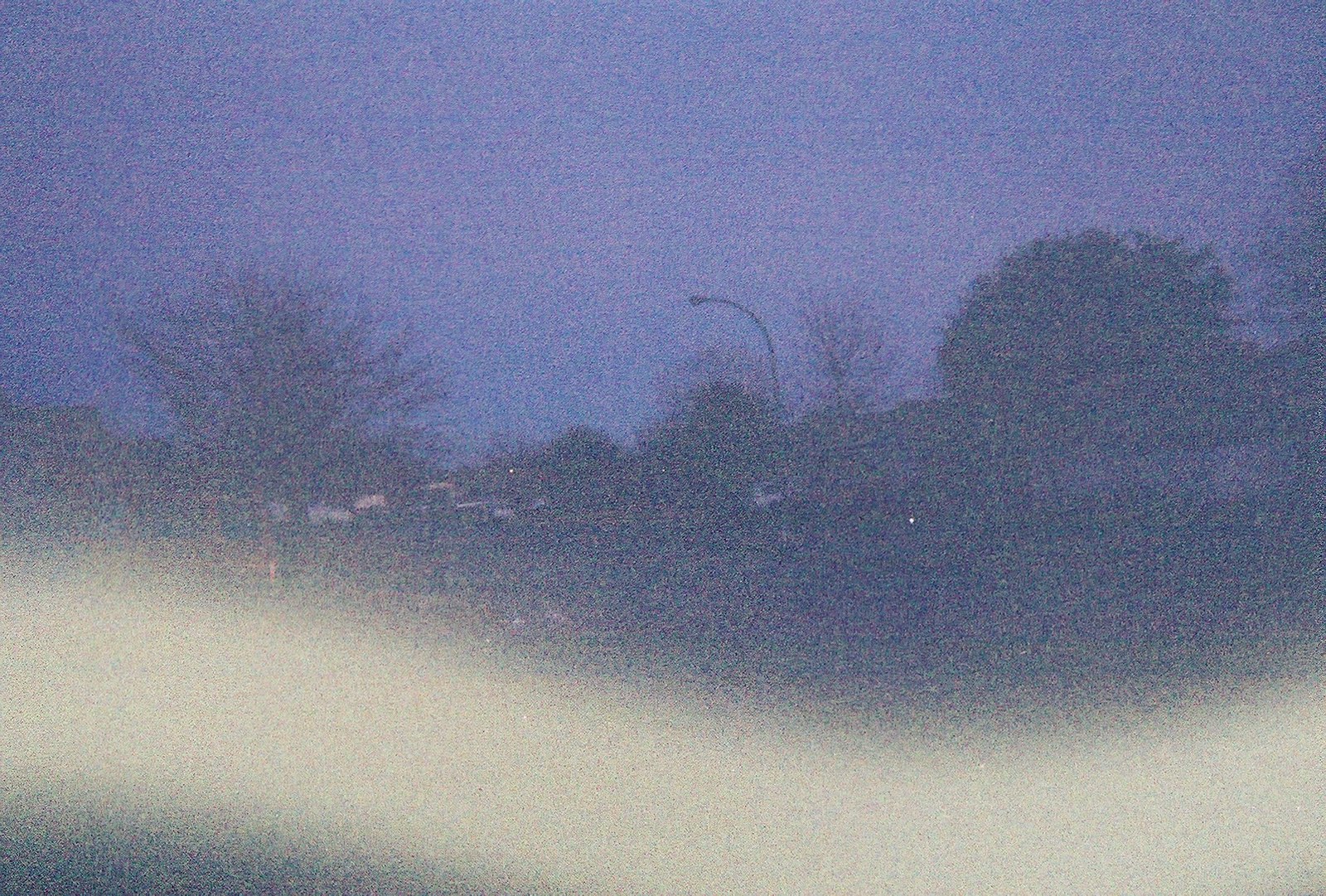A hazy and grainy outdoor photograph taken at dusk captures a moody, dimly lit neighborhood scene. The sky, enveloped in a dark, bluish hue, glows faintly as the sun sets. The horizon features several tree-like structures, with a noticeable barren, twiggy tree on the left side of the image, contrasting with a fuller, more rounded tree on the right. A curved streetlight with an unlit bulb stands prominently in the middle of the scene, adding a lonely focal point. The lower half of the photo is partially obscured by a wave of white mist or possibly a defect in the photo processing, creating an ethereal effect that obscures some details. The image evokes a sense of serene isolation, heightened by the mysterious white swath at the bottom.